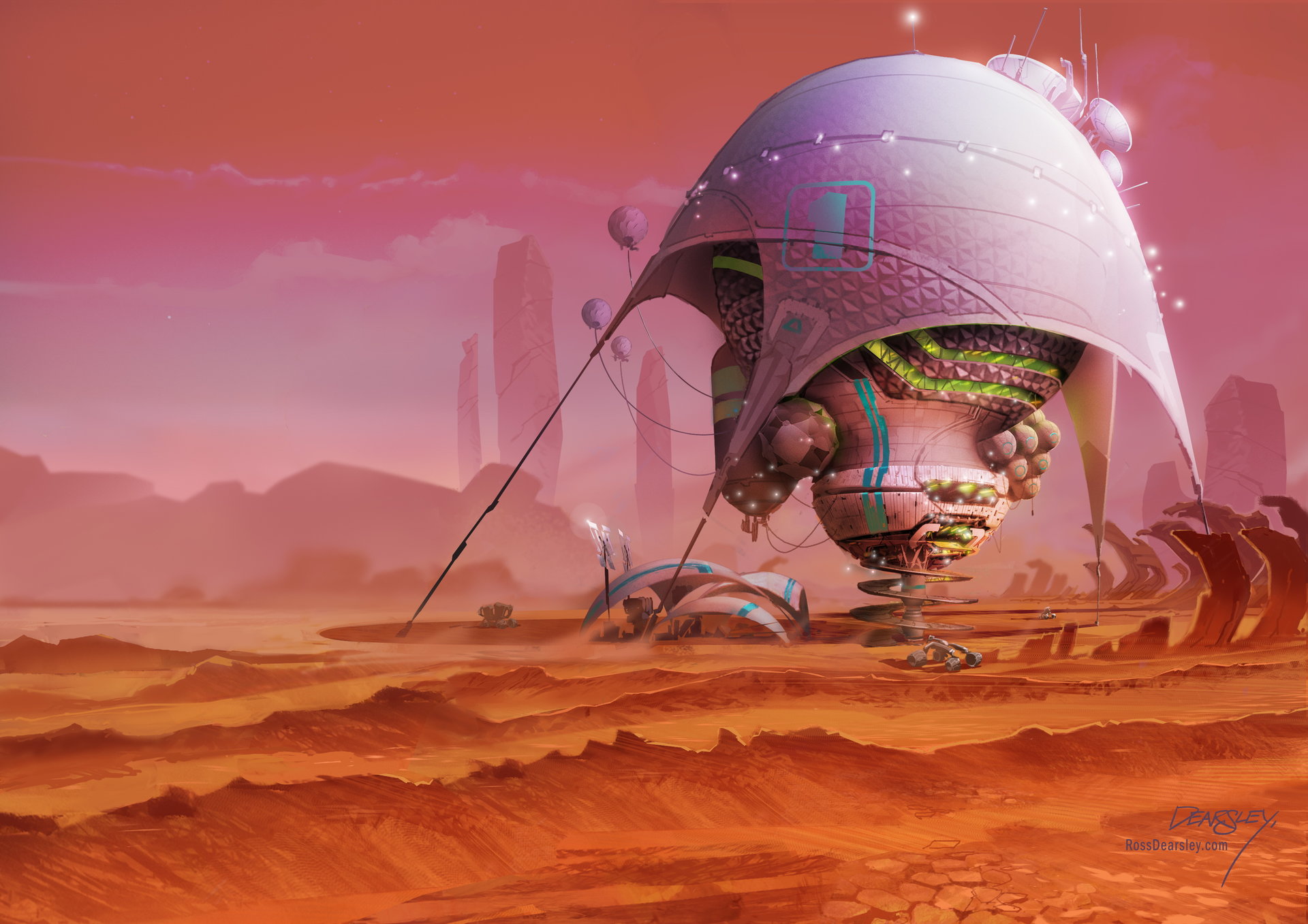The image is a detailed and imaginative sci-fi fantasy artwork set on what appears to be an alien planet, perhaps reminiscent of Mars. The canvas is horizontal and divided into two distinct color palettes. The sky occupies the top half, dominated by hues of pink intermingled with light orange, transitioning to deeper shades of pink and orange clouds. The ground in the lower half is primarily an orange and brown mix, adorned with light orange sands and darker orange, hilly mounds, creating a barren, rocky landscape.

In the background, a couple of skyscraper-like rock formations rise smoothly, bathed in soft pink and light orange hues, seamlessly blending into the sky. The central focus is a complex, alien structure situated slightly to the right of the image. This structure features a pink, light bulb-shaped building, which seems mechanical. It is partially covered by a light pink tarp or canopy, secured with wires on all four sides. 

The base of the structure resembles a spring or corkscrew, suggesting a possible mining operation. Adding to its intricate design are several small satellite dishes and turquoise and lime green lines that accent its silverish-pink surface. The overall scene is both otherworldly and detailed, evoking a sense of futuristic exploration on a distant, alien landscape.